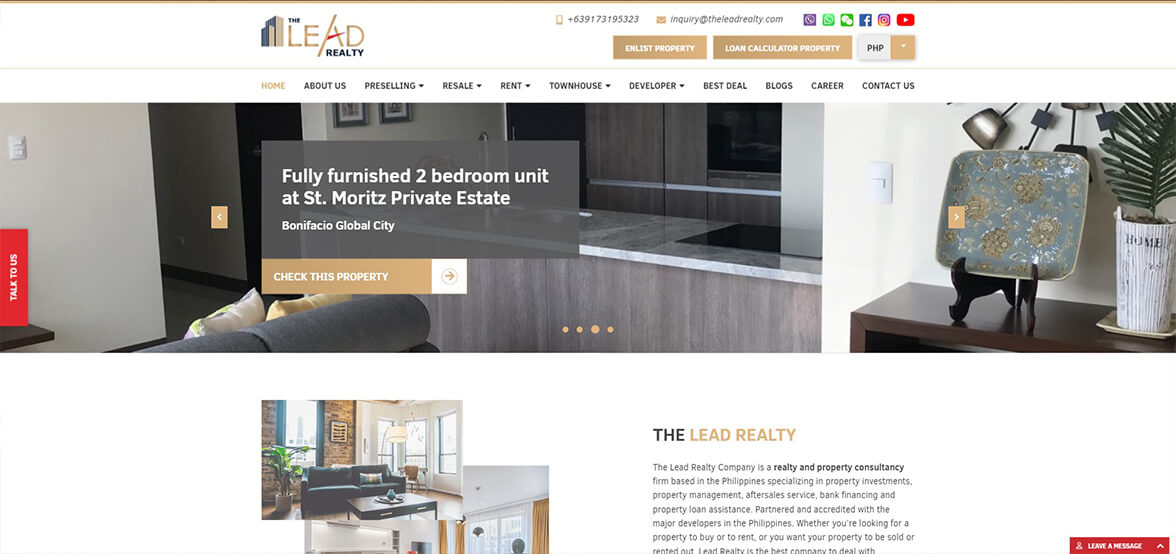The screenshot, taken from the website "The Lead Realty," shows a detailed and interactive property listing interface. In the upper section, there are various ways to contact the realty, including a prominently displayed phone number and a clickable email link. A visually striking button labeled "Enlist Property" is available, along with a "Loan Calculator" feature and a PHP button. 

At the top, a series of social media icons allows users to connect via platforms such as Facebook, YouTube, and Instagram. The central part of the interface showcases an image of a fully furnished living room that seamlessly extends into the kitchen area. Superimposed on this image, text highlights a "Fully Furnished Two-Bedroom Unit at St. Morris Private Estate," located in Bonifacio Global City. A call-to-action button labeled "Check This Property," accompanied by a white square with a right-pointing arrow, invites viewers to explore further.

To the right of the main image, another picture focuses on home decor elements such as a plant, wall decorations, and a fancy clay plate on a plate holder. Scrolling down, the viewer encounters additional images of comfortable living rooms. The footer of the page features the label "The Lead Realty" and includes a red-tagged area for visitors to leave a message.